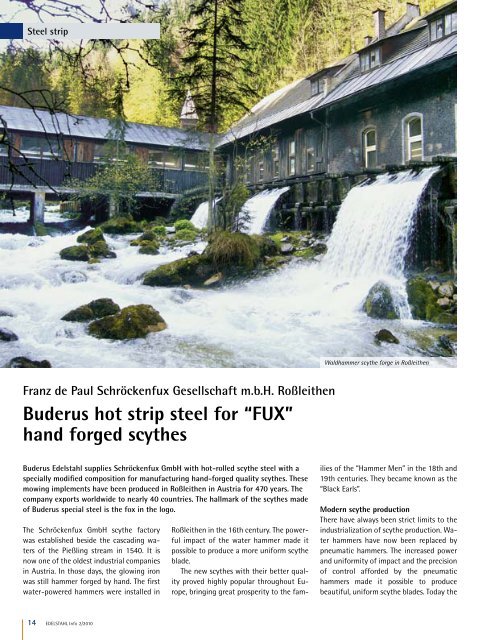This detailed descriptive caption amalgamates shared and emphasized details from all three captions:

The photograph, likely part of a magazine article or advertisement, showcases an outdoor scene featuring a large, grayish-blue, L-shaped building, reminiscent of a barn or house, set in a landscape that could be evocative of the Pacific Northwest. The structure, which appears to have windows and a metallic silver roof, is adorned with a distinct stone wall or fence on one side. From this wall, three prominent waterfalls cascade down into a turbulent, white-water river below, populated with moss-covered rocks that suggest a natural yet rugged environment. In the background of the image, there's another similar building visible amid a backdrop of trees, aligning perpendicularly to the main structure. At the bottom of the photograph, German text details an advertisement for "Buderus Hot Strip Steel" and "Hand Forged Sides," amongst other information, spread across approximately four paragraphs. The page is numbered 14, indicating its placement within the publication.